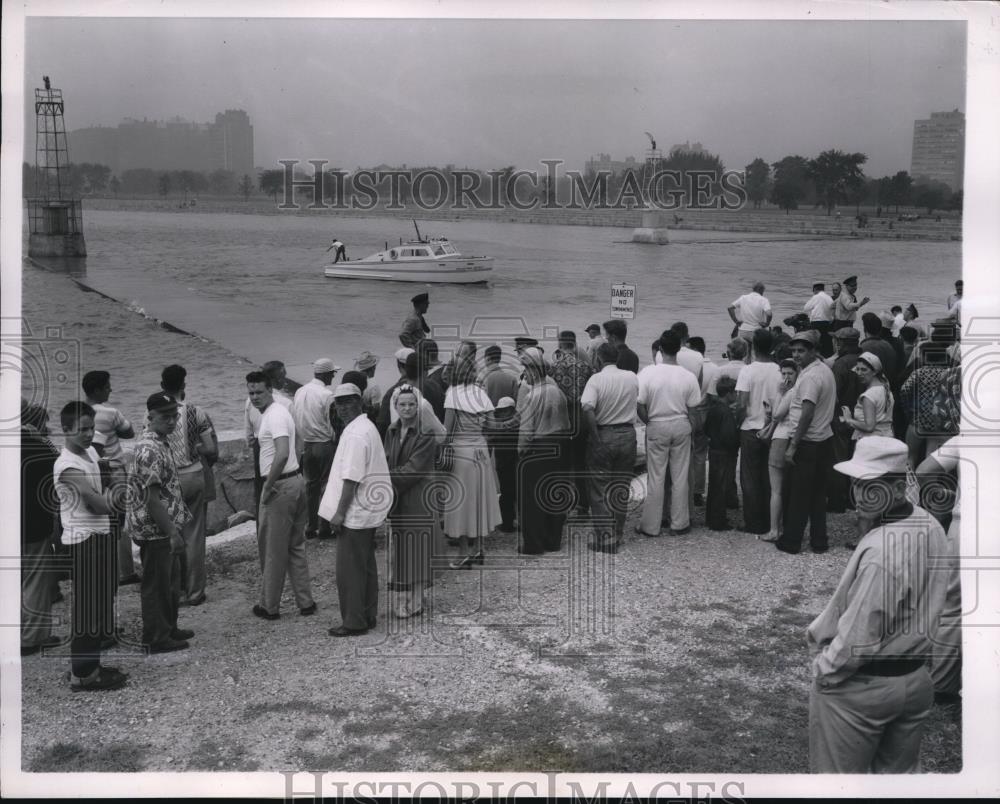This black and white press photograph from 1954 captures a dramatic dragging operation near Chicago, where authorities search the water for fishermen swept off a pier by rising tides. The image is watermarked with "historic images" at both the top and bottom. A significant crowd, mostly dressed in typical 1950s attire—white t-shirts, tank tops, and long skirts for the women—lines the shore, intently observing the operation. The crowd is mostly facing the water, though a few individuals turn towards the camera.

Visible in the scene are several boats, including what appears to be a police or fire patrol motorboat, maneuvering near the concrete pier where the dragging lines are in use. The operation is set against a city backdrop; high-rise buildings and trees are faintly visible through the haze. The pier itself features prominently, with concrete structures and a noticeable "danger: no swimming" sign. Officers in uniforms, suggesting the presence of law enforcement personnel, are seen holding back the gathered onlookers, adding an element of urgency and control to the scene. In the river, amidst the operation's activity, a man on the boat appears to be handling equipment, perhaps an anchor or net, involved in the search, while in the background, concrete stairs and other man-made structures punctuate the city's waterfront.